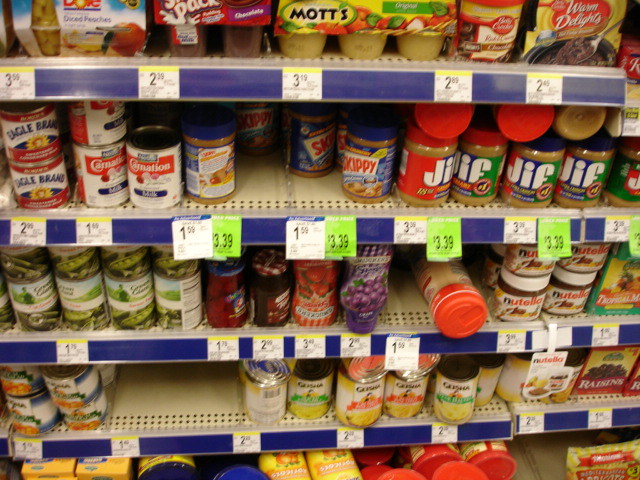This photograph captures the inside of a grocery store shelf from a front-facing angle, giving the perspective as if the viewer is standing and looking down at the shelves. Five visible shelves are stocked with a variety of items, each marked with white price tags displaying black numbers. The shelves are beige with perforations running horizontally along the edges, contrasted by a deep blue front lining.

On the top shelf, there are a variety of fruit products including diced peaches in small plastic containers, Mott's applesauce, Dole fruit cups, and chocolate pudding packs. Additionally, there are cans of Betty Crocker cake frosting and Warm Delights cake mix.

The second shelf features sweetened condensed milk, evaporated milk, and popular brands of peanut butter such as Skippy and Jif, along with Carnation condensed milk cans.

The third shelf holds an assortment of canned vegetables, various jams and jellies, and containers of Nutella spread. Below that, on the fourth shelf, there are more canned vegetables and possibly cans of tuna, along with boxes of raisins situated to the side on the right. The specific contents of the bottom shelf are not clearly visible. Each shelf edge is lined with small square white labels indicating the prices of the displayed items.